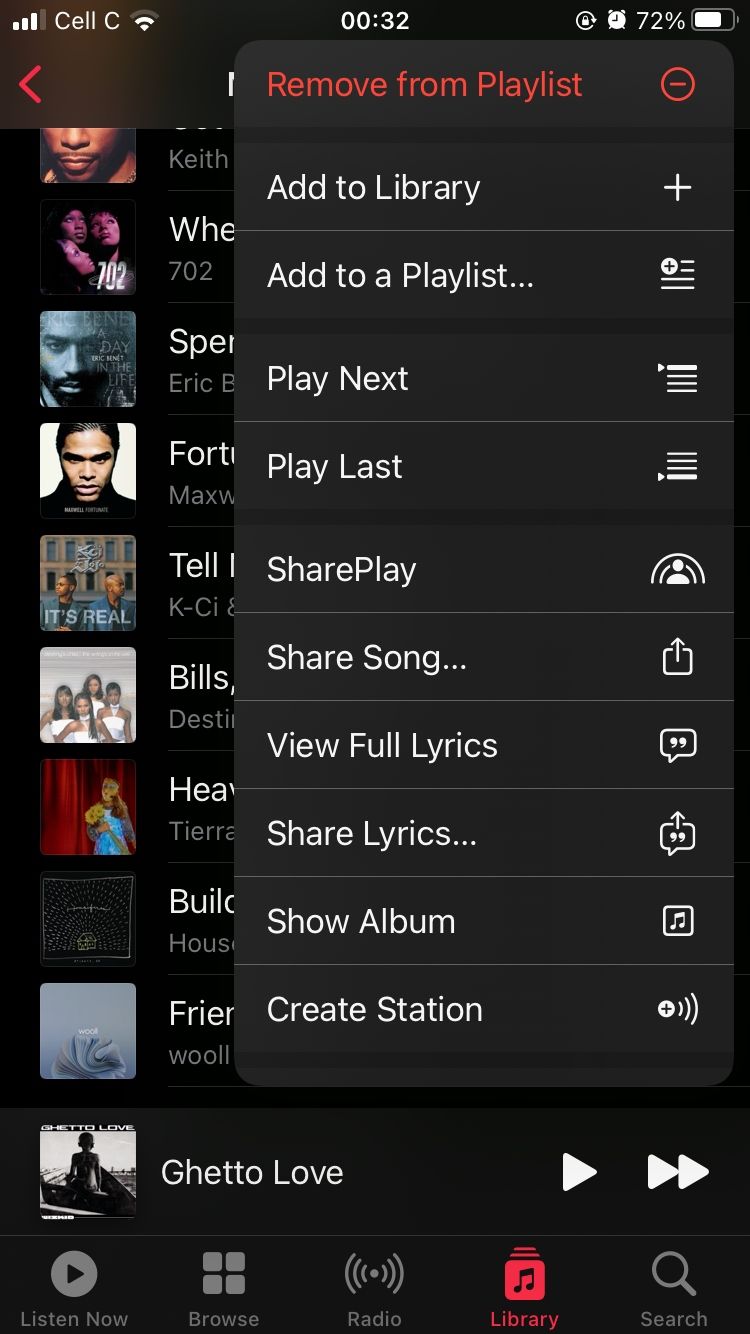A screenshot from a mobile phone displays various elements of the device's status and a detailed pop-up menu. At the top, the status bar shows a mobile signal icon with three out of four bars, indicating moderate signal strength. Next to it, the carrier name "Cell C" is displayed in white font, followed by a Wi-Fi icon with two out of three bars, suggesting a decent Wi-Fi connection. The time is shown as "00:32". Further along, an SD card icon, an alarm clock icon, and a battery percentage of "72%" are visible, alongside a battery icon.

Below the status bar, a pop-up menu appears. The top portion of the menu is gray, featuring the option "Remove from playlist" in red font, accompanied by a red circle with a minus sign. The subsequent options, listed in white font, include: "Add to library", "Add to playlist", "Play next", "Play last", "Share play", "Share song", "View full lyrics", "Share lyrics", "Show album", and "Create station". Each option is paired with an icon to its right: starting at the top, there's a plus icon next to "Add to library", and both "Add to playlist" and "Play next" are marked with multiple lines icons, continuing in similar fashion for the other options.